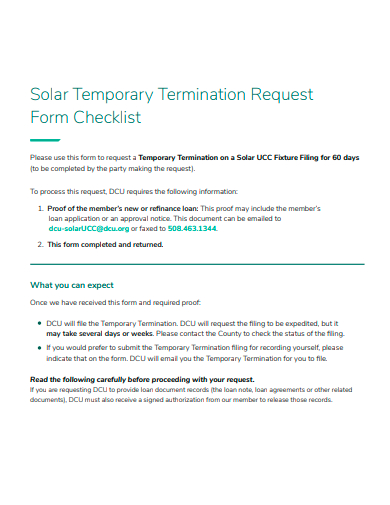A screenshot of the "Solar Temporary Termination Request Form Checklist" is displayed. The header, in teal, reads "Solar Temporary Termination Request Form Checklist" with a matching teal dash-line below it. The checklist contains four or five bullet points, detailing the steps or requirements for the temporary termination process. The background of the form is white, and the primary text is black, ensuring clear readability. Additional important information is highlighted in bold, teal font, with a notable section at the bottom titled "What You Can Expect," also in bolded teal, indicating a summary or detailed explanation of subsequent steps following the form submission. The color scheme and layout suggest a structured and user-friendly document for users seeking to temporarily terminate their solar service.